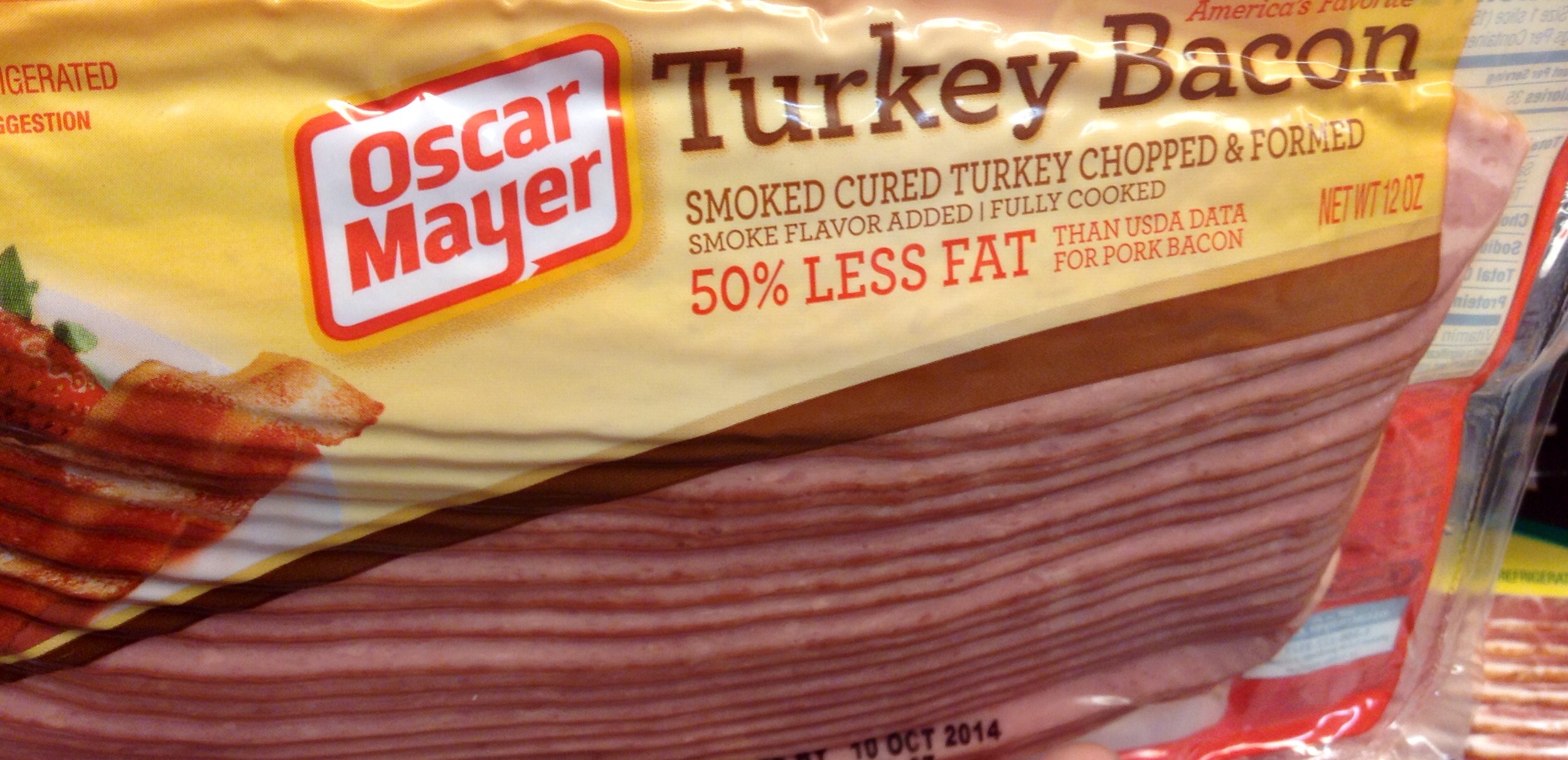The image features a package of Oscar Mayer Turkey Bacon. In the top left corner, there is a prominent yellow section. Centrally, a silica white square is bordered in red with red text that reads "Oscar Mayer." Above the logo, it states "Turkey Bacon," and below it, the package describes the product as "Smoked Cured Turkey Chopped and Formed, Smoke Flavor Added, Fully Cooked." Further down, the packaging highlights "50% Less Fat," comparing it to USDA data for pork bacon, and specifies that the package weighs 12 ounces. To the left of the text, there is an image of cooked turkey bacon strips, illustrating the product. Below this, a stacked pile of turkey bacon strips is visible. Near the bottom, the packaging indicates the expiration date as "October 2014." On the far left side, part of another package's label is partially visible, providing a glimpse of the back or side label of the turkey bacon package.